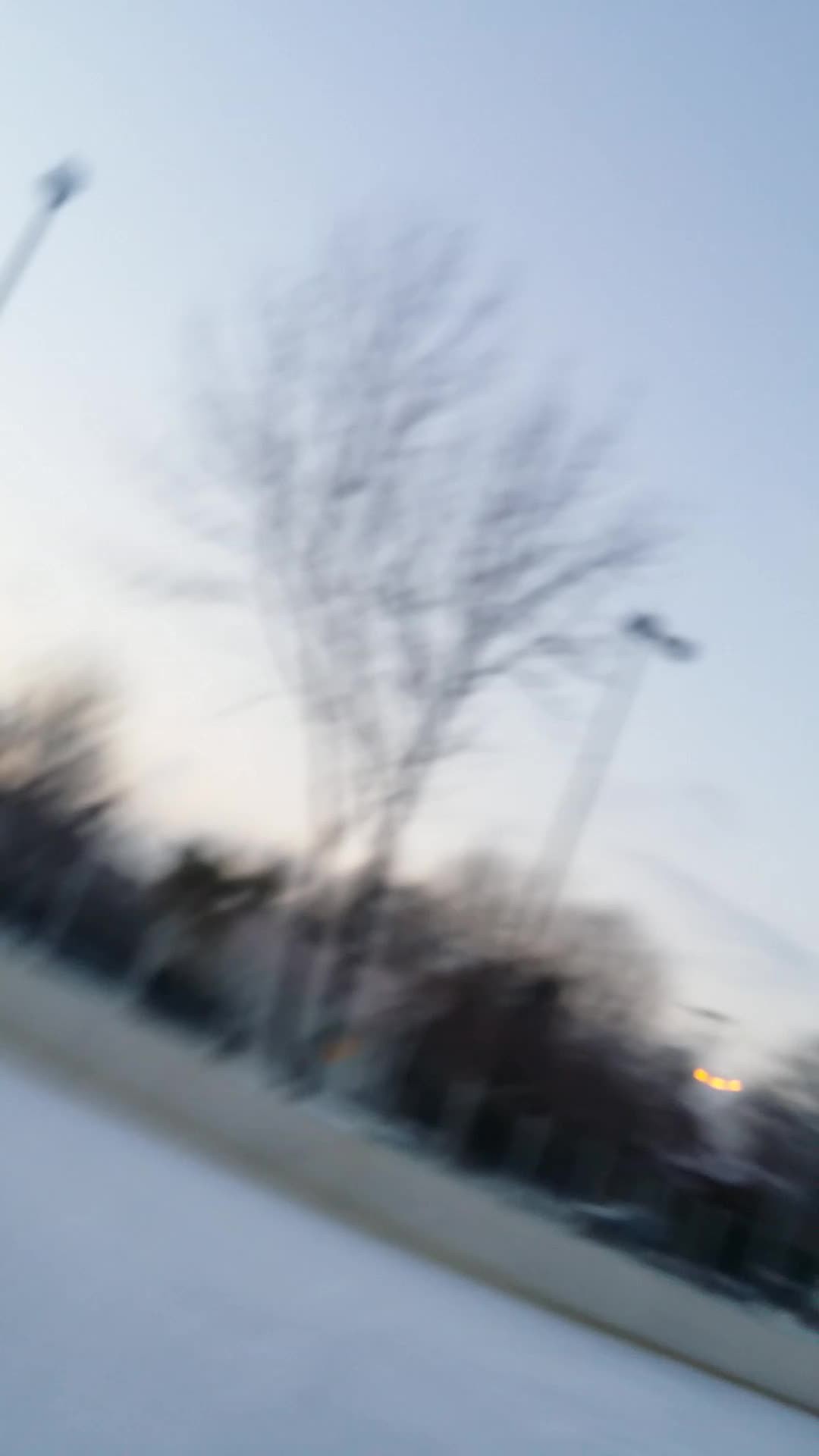The tilted, blurry image appears to be taken outdoors during what might be sunrise, given the faint orange streak in the sky and the overall brightness. The setting is snowy with a low retaining wall that supports leafless trees and potentially an electrical utility box positioned on the right side. Scaffolding can be faintly discerned in the background. The sky has a grayish hue with hints of blue, and prominent street pole lights are visible, though they are not illuminated. Dark-colored buildings are situated near the bottom of the image, interspersed with at least one light-colored structure. The photograph's diagonal orientation adds to its obscurity, with various dark and white elements near the lower section that could be part of the snow, a dashboard, or other objects.